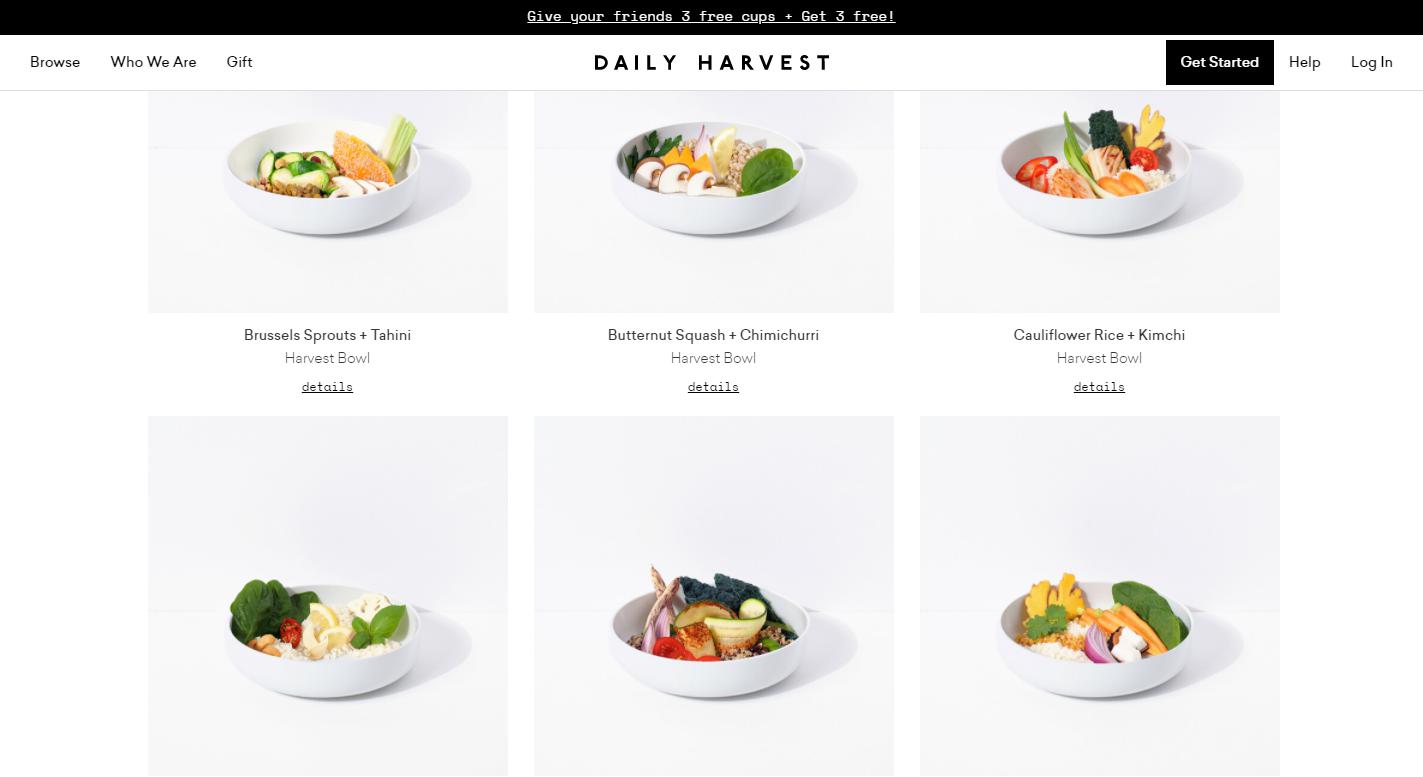The image depicts a screenshot of the Daily Harvest website, prominently featuring their logo in the center. Above the logo, there's a promotional banner stating "Give your friends 3 free cups and get 3 free," indicating a referral program. 

To the left of the screen, a navigation menu displays options labeled "Browse," "Who We Are," and "Gift." On the right, options include "Get Started," "Help," and "Log In." 

Below the navigation bar, the website showcases six images of food items, three of which are only partially visible. Each fully visible image includes a description: 
1. "Brussels Sprouts in Tanny Harvest Bowl" with a clickable button for more information.
2. "Butternut Squash in Chimichurri."
3. "Cauliflower Rice in Kimchi."

This section suggests that Daily Harvest offers a variety of prepared meals or meal kits, featuring dishes that potentially include a mix of global flavors. The primary focus seems to be on providing convenient and healthy meal options that users can prepare at home.